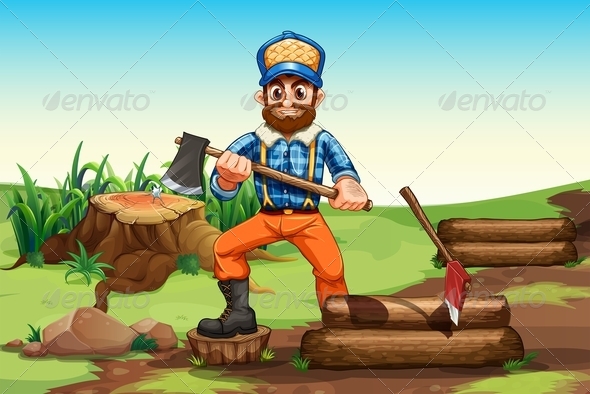The cartoony image depicts a lumberjack with a distinctive and detailed appearance. The man has a bushy brown beard and mustache, bushy brown eyebrows, and brown eyes. He wears a cap that is blue with a tan front adorned with an axe pattern. His attire includes a blue plaid shirt, tan suspenders connected to a black belt, and orange pants. He also sports tall black boots, one of which rests on a tree stump while the other is obscured by logs. Notably, his hands are covered in hair. He holds a red-headed axe firmly in his large hands. Beside him lies a pile of logs with another axe embedded in them, and another larger tree stump is visible behind him. The background includes patches of grass, and the entire scene is interspersed with the word "Envato," forming a diamond pattern across the image.